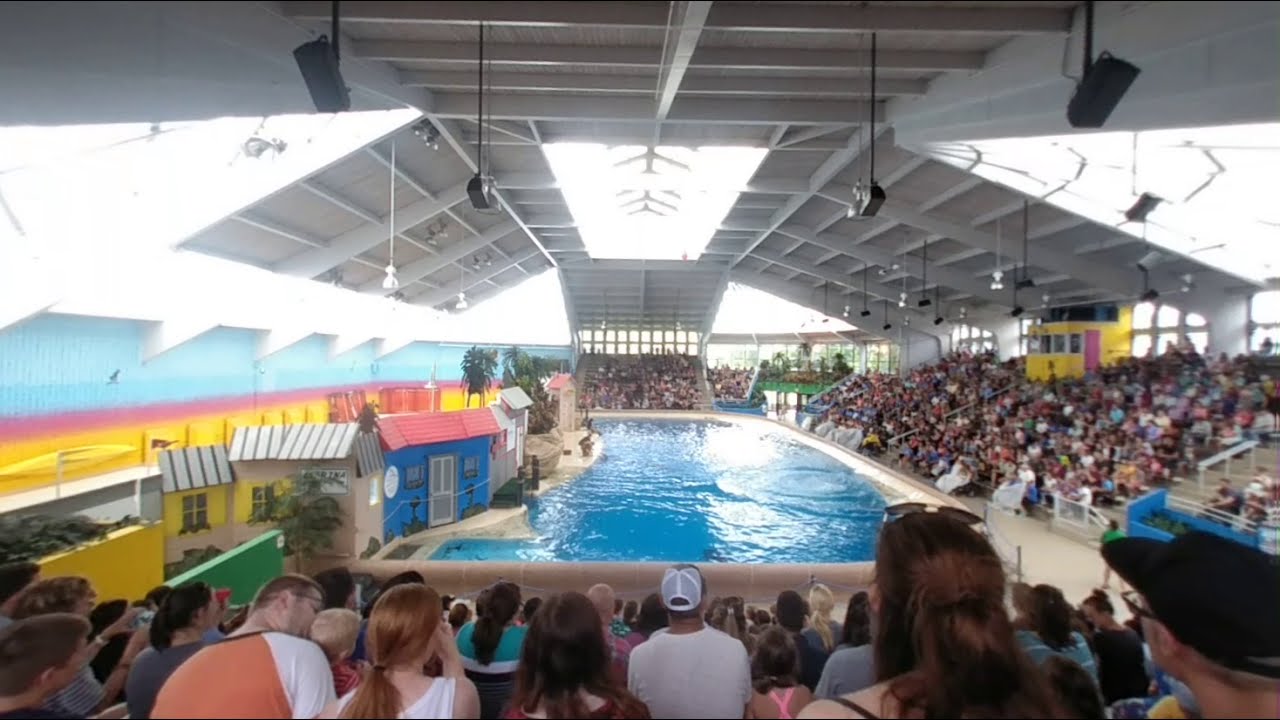This is a detailed, horizontal rectangular photograph taken with an unusual lens, depicting a bustling pool area with a semi-outdoors, partially covered ceiling. The scene captures a large crowd, with people seated in the foreground and along the right side on bleacher seats, all intently watching the center of the image where a pool is located. The left side features a staged, mock beach front area adorned with small structures resembling houses or snack bars, painted in vibrant hues of blue, yellow, and roofs of various colors such as red and white with green stripes. The background reveals additional bleachers filled with spectators. Bright light streams in through skylights, enhancing the atmosphere of an event or show taking place near the water. The image is rich in colors including gray, white, light blue, purple, pink, yellow, orange, and black, but contains no visible text, focusing entirely on the lively setting and its audience.